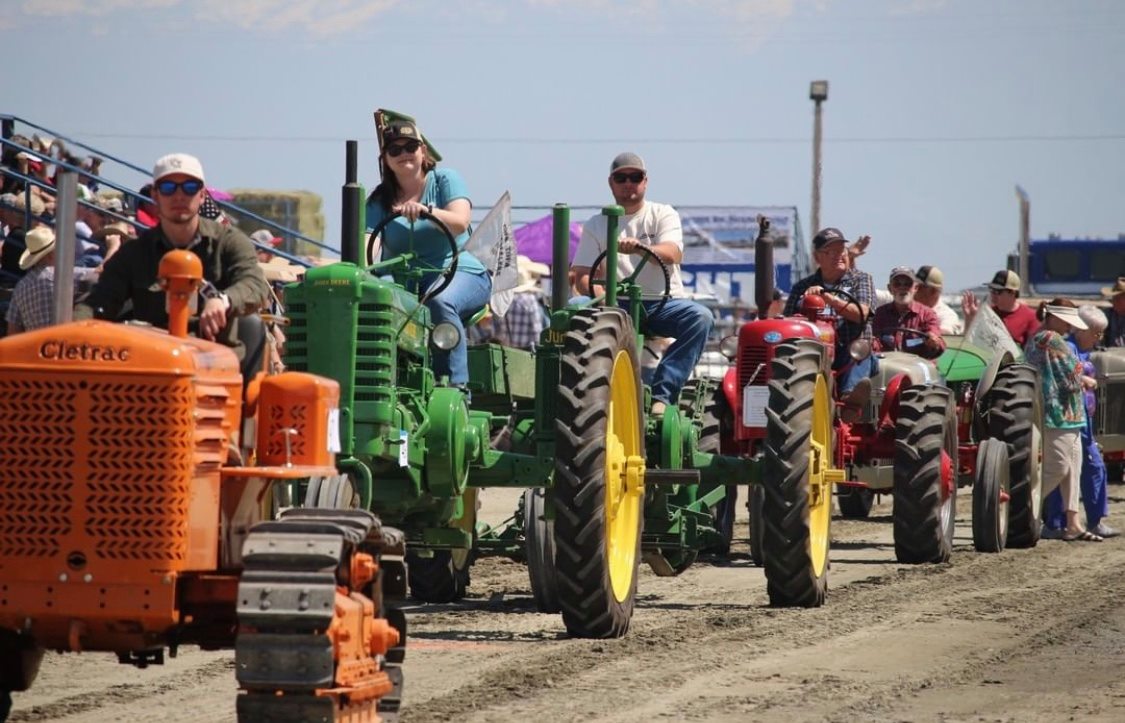This vibrant color photograph captures a lively scene at a state fair, where a parade of vintage tractors is progressing along a dirt road adjacent to stadium seating filled with spectators. The sky is bright and sunny with a few clouds, accentuating the festive atmosphere. Leading the procession is a young man in a sideways ball cap and mirror sunglasses, driving a bright orange Cle-Trac tractor with distinctive track wheels. Behind him is a woman in a blue outfit and pirate-style kerchief, perched on a tall John Deere tractor painted in signature green with yellow wheels. Following her, there's a man in a white shirt and blue pants on another green John Deere tractor. Further back, an older man wearing a flannel shirt and military-style hat drives a red tractor, possibly a Farmall, trailed by a red-shirted man on another green tractor with an additional white-shirted passenger. The lineup of tractors includes a variety of colors—orange, green, and red—mirroring the diversity of the participants' apparel, many of whom don hats or baseball caps. Spectators can be seen in the stands, with sponsorship banners and stadium lights in the background, enhancing the sense of an organized and well-attended event. Two women can also be seen walking on the dirt path towards the field, contributing to the bustling activity of the fairgrounds.